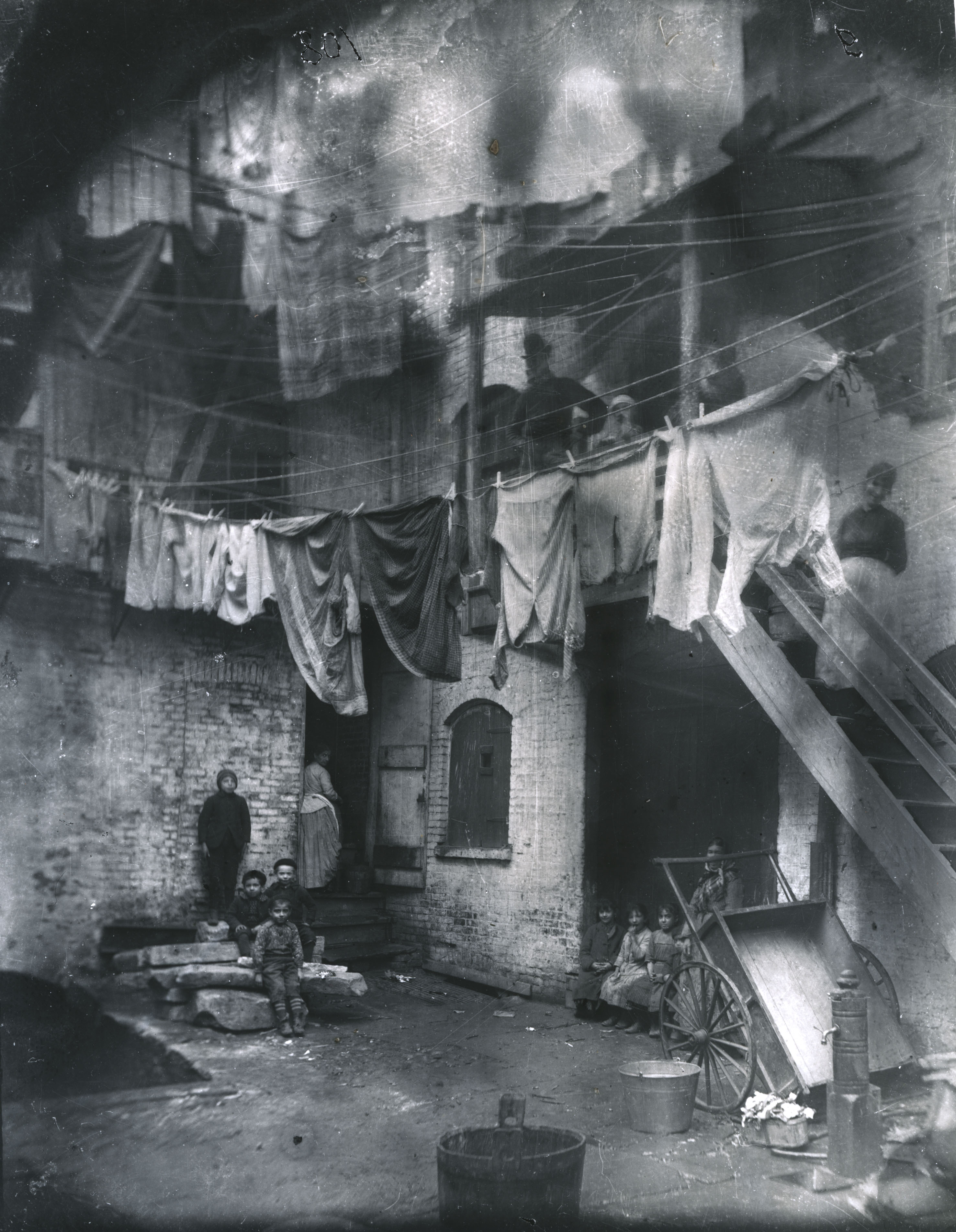This black-and-white photograph, likely from the early 1900s to 1930s, depicts a scene in a tenement courtyard of a very poor neighborhood. The brick buildings, spanning at least three stories, frame the bustling courtyard where life unfolds amidst evident poverty. 

Children, dressed in overalls and long dresses, sit on rocks against a brick wall. Nearby, a person—possibly a woman or an older child—in black attire and a headscarf stands solemnly. To the right, a woman in a long dress with a white apron stands in a doorway, while an alcove further along houses three more children and an adult. An old wooden wagon with large wheels rests on the dark cement floor beside two wash tubs.

The scene is further animated by multiple clotheslines, heavy with garments, stretching between balconies and across various levels of the buildings. Women can be seen ascending the stairs to higher floors, engaged in their daily routines. On one of the upper floors, a man in a black outfit and top hat overlooks the courtyard, adding to the sense of a tight-knit yet struggling community.

Overall, the image captures the stark realities of urban poverty, with every detail—the clothing, the makeshift furniture, and the communal spaces—telling the story of the tenement dwellers' efforts to maintain some semblance of normalcy amid hardship.